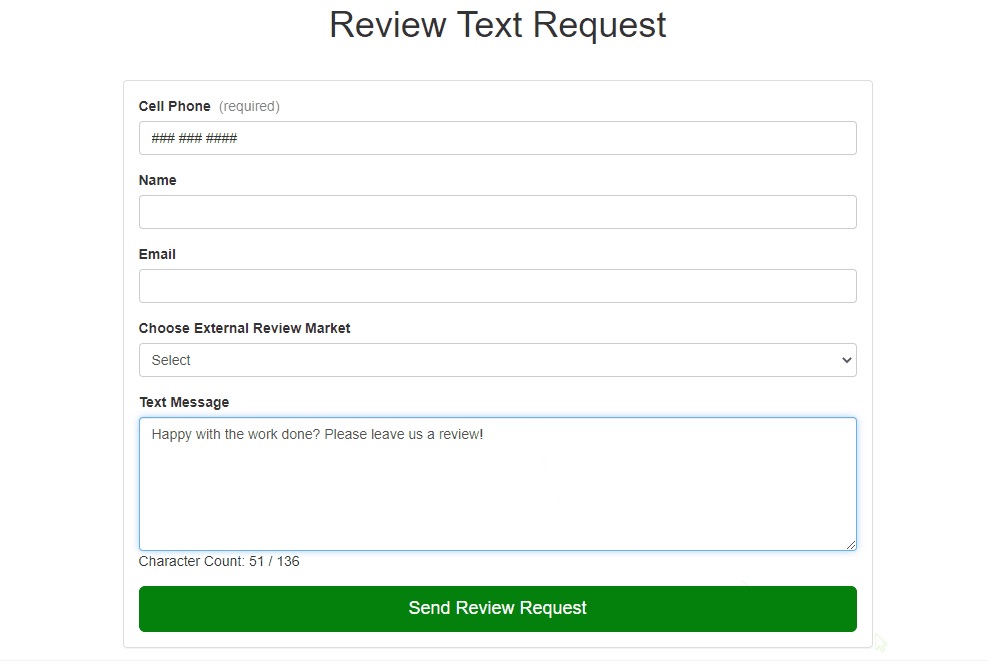The image is a screenshot of a computer screen showing a "Review Text Request" form. At the top of the page, the title "Review Text Request" is prominently displayed. Below this title, several input fields are present:

1. **Cell Phone** (Required): Users must enter their cell phone number in this field.
2. **Name**: An optional field for users to enter their name.
3. **Email**: An optional field for users to enter their email address.
4. **Choose External Review Market**: A drop-down menu for selecting the appropriate review market.

Further down the form, there is a text message composition area with a character count limit. In this screenshot, the user has written the following message: “Happy with the work done? Please leave us a review.” The character count indicates that 51 out of the maximum 136 characters have been used.

At the bottom of the form, a large green button labeled "Send Review Request" spans the width of the page. This button is designed for users to submit their completed review request.

Based on the content of the message asking if the user is "Happy with the work done," it is likely that this form is used by a company to collect reviews for their services.